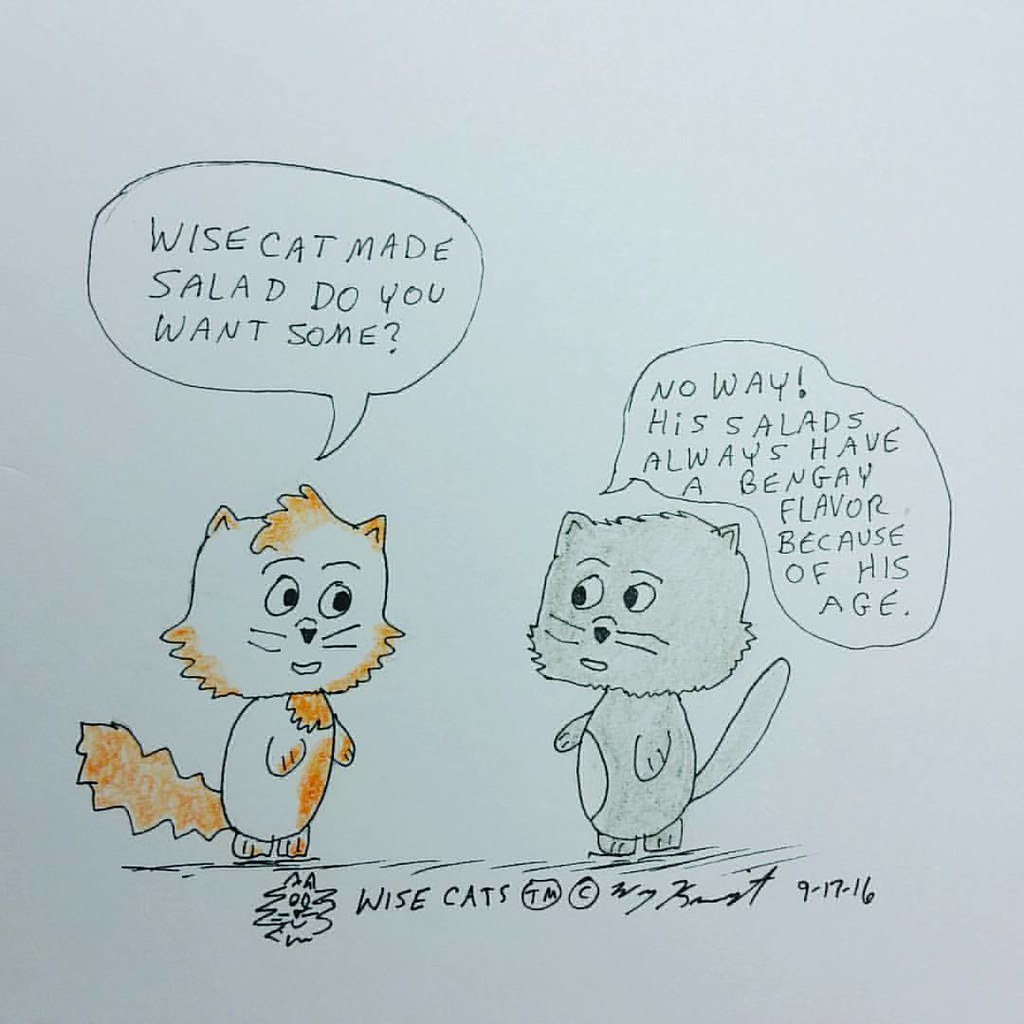This hand-drawn comic titled **"Wisecats"** features two cartoon cats standing upright on their hind legs, engaging in a humorous conversation about salad. The left cat, with a white coat and orange spots, and an orange tail, holds a speech bubble that says, "**Why's cat made salad? Do you want some?**” In response, the gray cat on the right, which has a white belly, replies "**No way, his salads always have a Bengay flavor because of his age.**" The scene is set against a solid white background, with the characters and their speech bubbles centrally positioned. Below the cats is the text "**Wisecats TM copyright**," along with the artist's signature and the date "**9-17-16**." Additional details include black marker shading at the cats' feet, indicating they are standing on a solid surface, and a small scribbled cat head near the trademark text. The colors are primarily off-white, black, orange, and gray, giving the comic a classic, newspaper-strip feel.